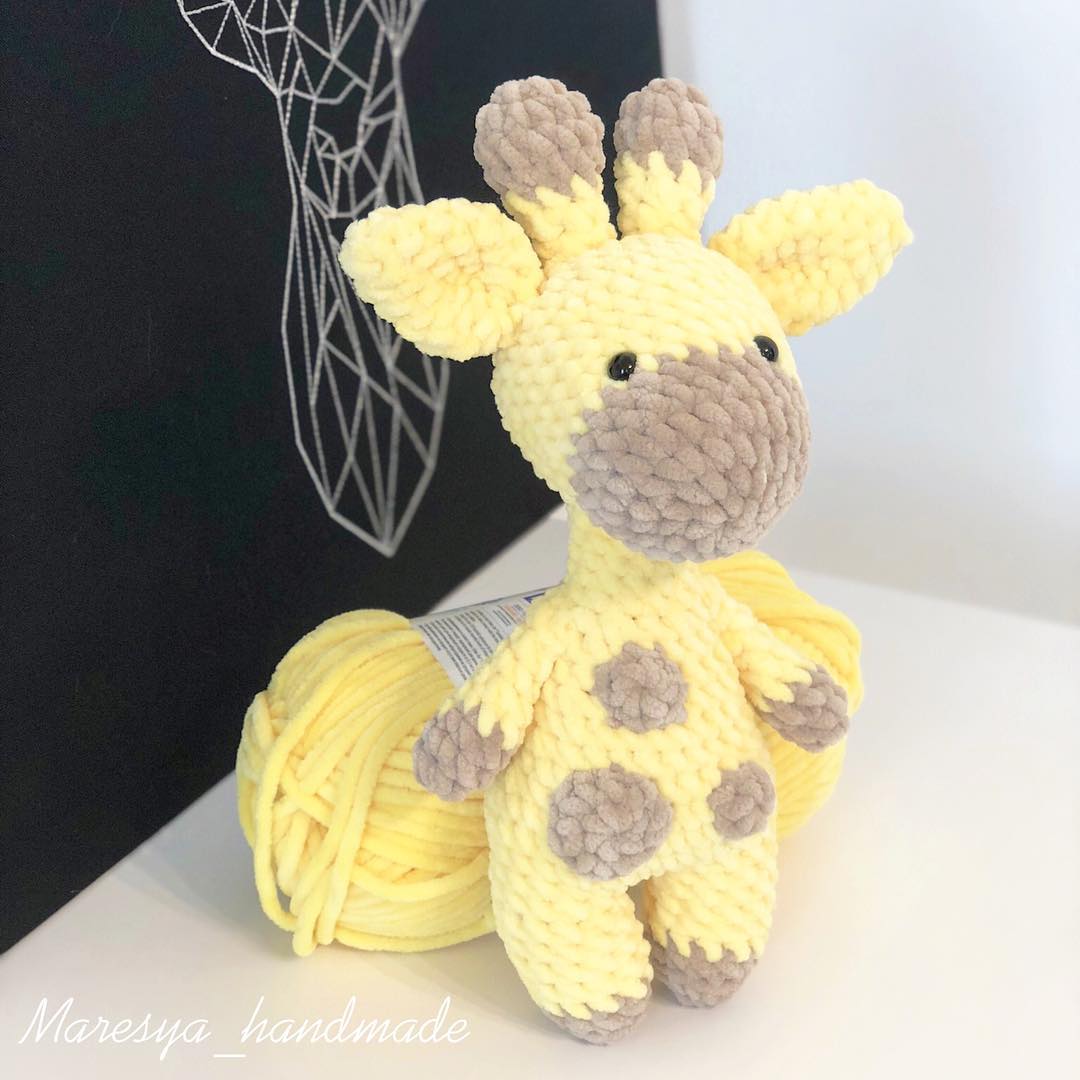This detailed and high-quality photograph captures a hand-crocheted giraffe stuffed animal, made primarily of yellow yarn with taupe-brown accents. The adorable giraffe, standing upright and slightly leaning against a full skein of the same yellow yarn, showcases fine craftsmanship. It features brown tips on its ears, horns, and limbs, with brown spots adorning its body. The giraffe's endearing expression is completed by its small black glass eyes. The background presents a stark contrast with a white surface on one side and an abstract drawing on a black surface on the other. In the lower left corner, the creator's name "Mareska Handmade" is elegantly displayed, highlighting the brand behind this charming creation.